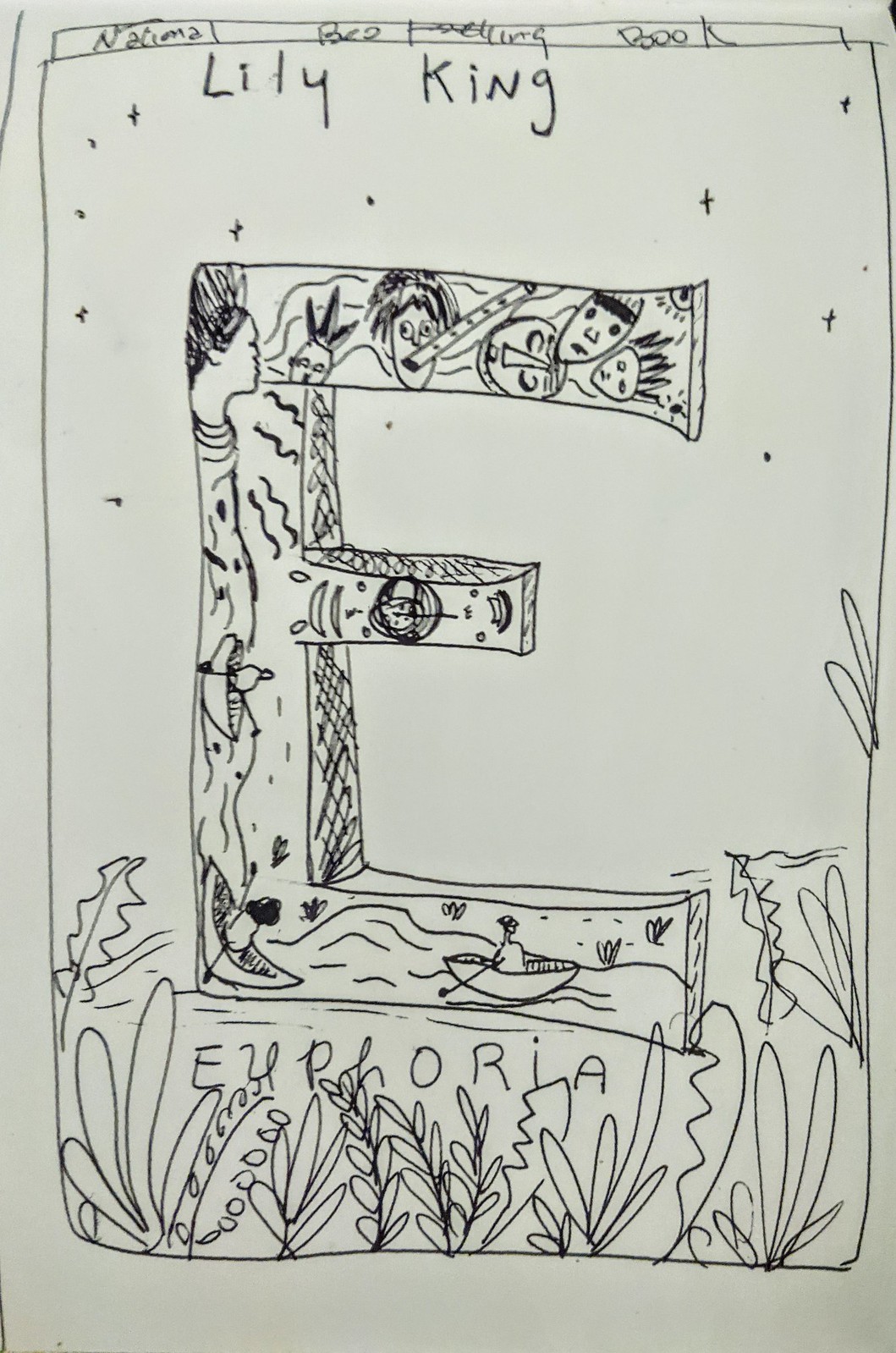Photograph of a detailed black-and-white drawing on white paper. The image is vertically oriented and bordered by a black frame. At the top, the text "Lily King" is prominently displayed in black lettering. Below this, the word "Euphoria" is inscribed in a smaller font. Both texts are positioned above the main focus of the drawing—a large, intricately designed letter 'E' situated in the center.

The letter 'E' itself is adorned with a variety of intricate elements. Within its contours, multiple faces are sketched, conveying different expressions. The lower part of the 'E' depicts a serene water scene featuring people paddling in canoes. Additionally, tiny cross-like shapes meant to represent birds are scattered around the letter 'E,' adding a sense of liveliness to the composition. The bottom section of the drawing includes representations of plants, grounding the elaborate design with a touch of nature.